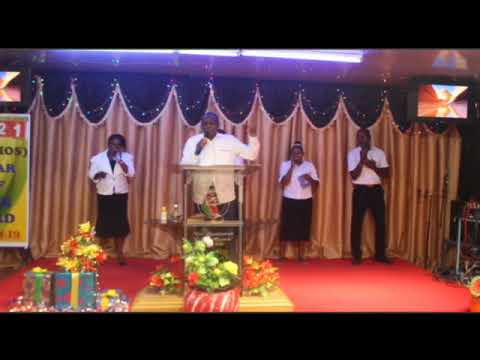The image depicts a vibrant scene at an African-style church during what seems to be a religious sermon. The stage is covered in a rich red carpet, and at the forefront stands a preacher at a clear acrylic or glass podium with a light tan wooden base. This preacher, dressed in a distinctive African-style shirt and hat, holds a microphone in his right hand and gestures with his left, suggesting he is preaching or singing.

In front of the podium, variously wrapped presents — including a blue one with a red ribbon and a silver one with a green ribbon — are surrounded by colorful potted plants with red, white, and yellow flowers. To the left of the podium, there is a table also adorned with floral decorations.

Behind the preacher, at least three people stand in a row, potentially participating in the service. These individuals are all dressed in white shirts; the two women on the left wear black skirts, the young man to the right dons black pants, and another man in blue jeans can be partially seen. A striking golden curtain with a curvy draping pattern and black trim, possibly topped with white, serves as a backdrop. Additionally, there is a television mounted on the top right of the wall and an unreadable sign on the left. The entire setup exudes a welcoming and festive atmosphere appropriate for a communal religious gathering.